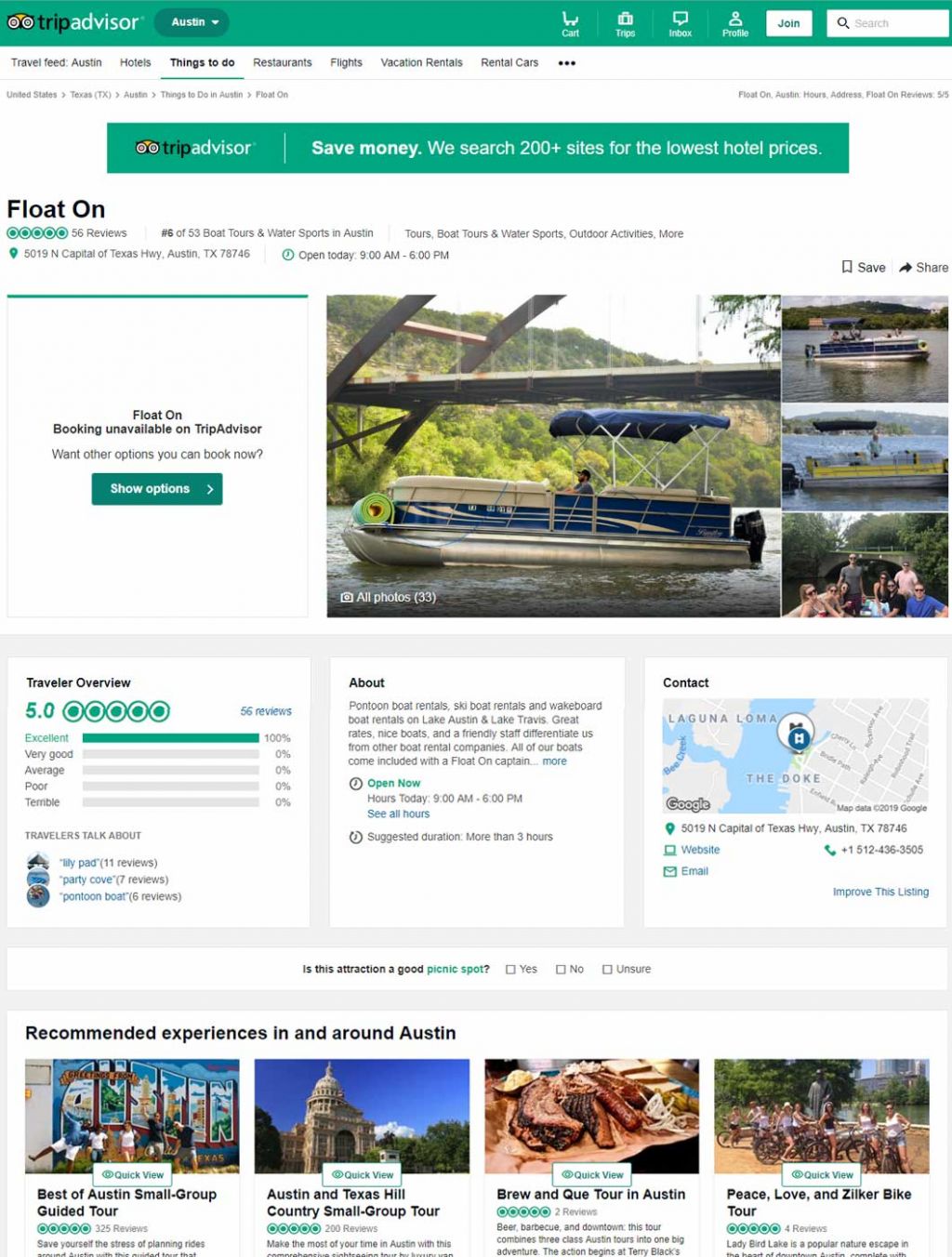The image is a screenshot of the TripAdvisor website, featuring a prominent green border at the top. Located in the upper left corner, the TripAdvisor logo, resembling two eyes, is distinctly visible. To its right appears a drop-down menu labeled "Austin," followed by a search bar and a "Join" button.

Below, a navigation menu is shown, with the "Things to Do" option highlighted and underlined in green. Directly beneath this menu is a green banner stating, "TripAdvisor saves you money. We search 200+ sites for the lowest hotel prices."

In the main content area, there is a photograph of a boat on a tranquil body of water. To the left of the image, text reads "Float On," with a note that booking is currently unavailable on TripAdvisor, and visitors are encouraged to explore other options. A prominent green button labeled "Show options" is available for users to click.

At the bottom of the screen, a series of three informational boxes is displayed. The first box, titled "Traveler Overview," boasts a 5.0 rating. The subsequent boxes are labeled "About" and "Contact with Map." 

Finally, at the very bottom, there is a section titled "Recommended Experiences in or around Austin." This section features four images accompanied by titles: "Best of Austin Small Group Guided Tour," "Austin and Texas Hill Country Small Group Tour," "Brew and 'Cue Tour in Austin," and "Peace, Love, and Zilker Bike Tour."